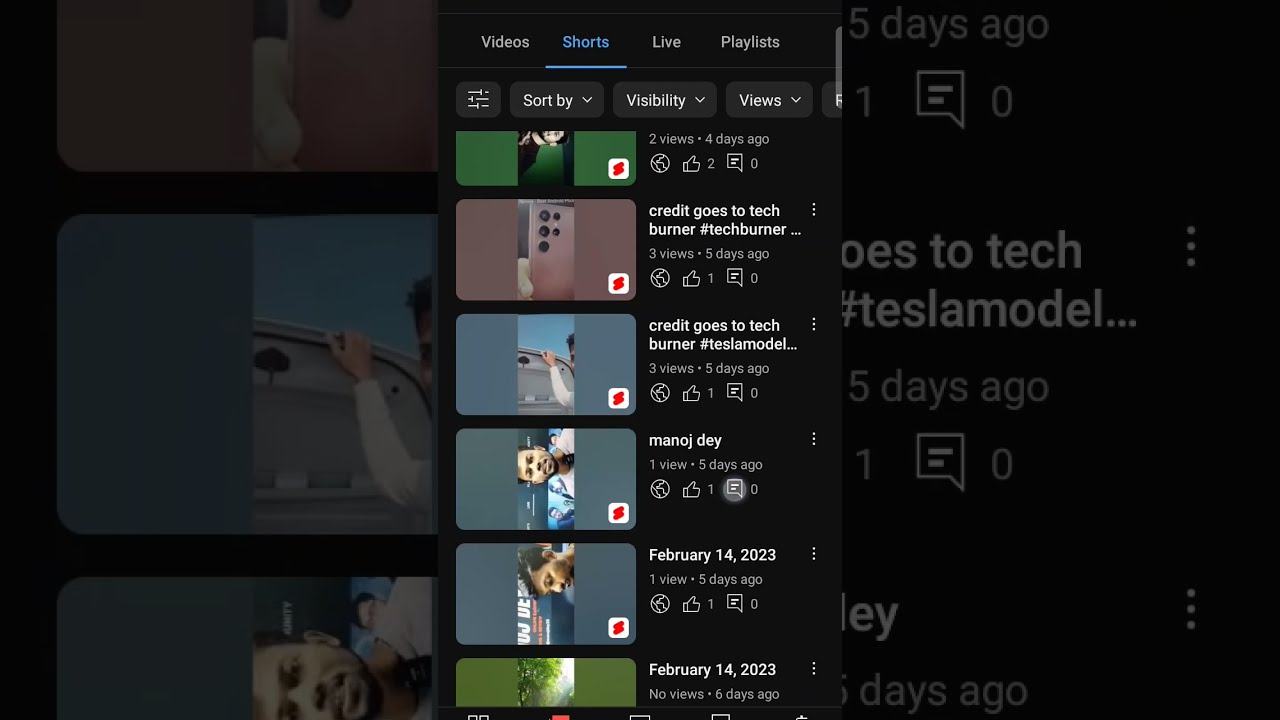This image appears to be a vertical screenshot from a phone displaying the YouTube interface, specifically focused on the Shorts tab. At the top, the tabs "Videos," "Shorts," "Live," and "Playlists" are visible, with "Shorts" highlighted in blue, indicating it is selected. Below these tabs are options labeled "Sort By," "Visibility," and "Views." 

The central part of the screen features a strip of six rectangular thumbnails arranged vertically on the left. Each thumbnail includes a still image from different YouTube Shorts. On the right side of each thumbnail, there are video titles in white text, view counts, and the duration elapsed since they were uploaded. The thumbnails include various subjects, such as a male with brown hair in two of the thumbnails and a camera on the back of a phone on another, all set against a black background.

Additionally, some video details and creator credits are visible, for instance, "2 views, 4 days ago" with a credit to "TechBurner" and "3 views, 5 days ago" accompanied by a few captions and dates. The outer sections surrounding this middle display are darker, emphasizing the vertical format of the screenshot.